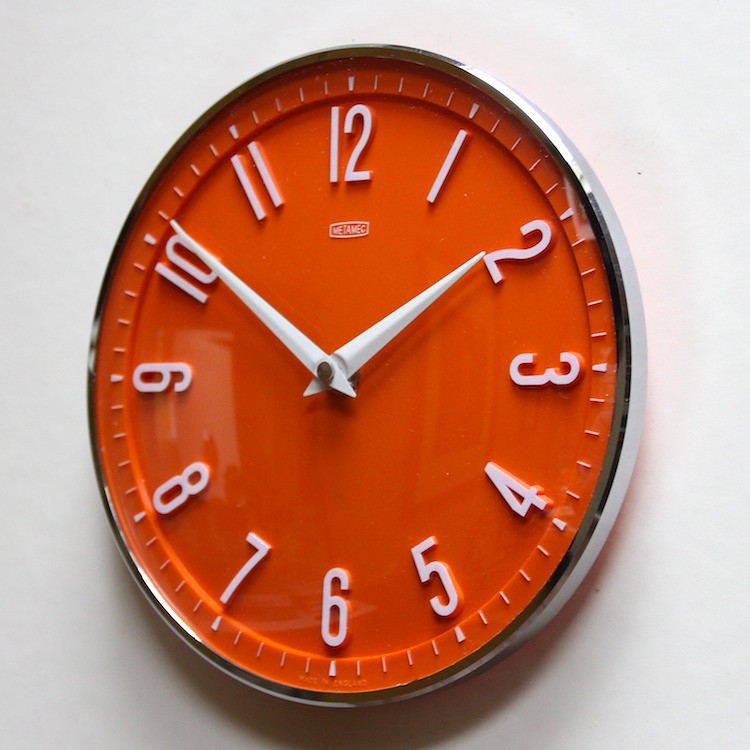The image features a red clock with prominent white numbers and pointers, mounted against a gray, ombre-effect background that transitions from lighter to darker shades at the corners. The clock, marked with "MetaMet" at the top and "Made in England" subtly at the bottom, is encased in a shiny silver rim that reflects light and surroundings. The red ceramic face includes white numerals (12, 1, 2, 3, 4, 5, 6, 7, 8, 9, 10, 11) and minute tick marks. The white hour and minute hands are bolted at the center, indicating a time of approximately 1:51. Shadows cast by the clock enhance the depth and contrast of the background.